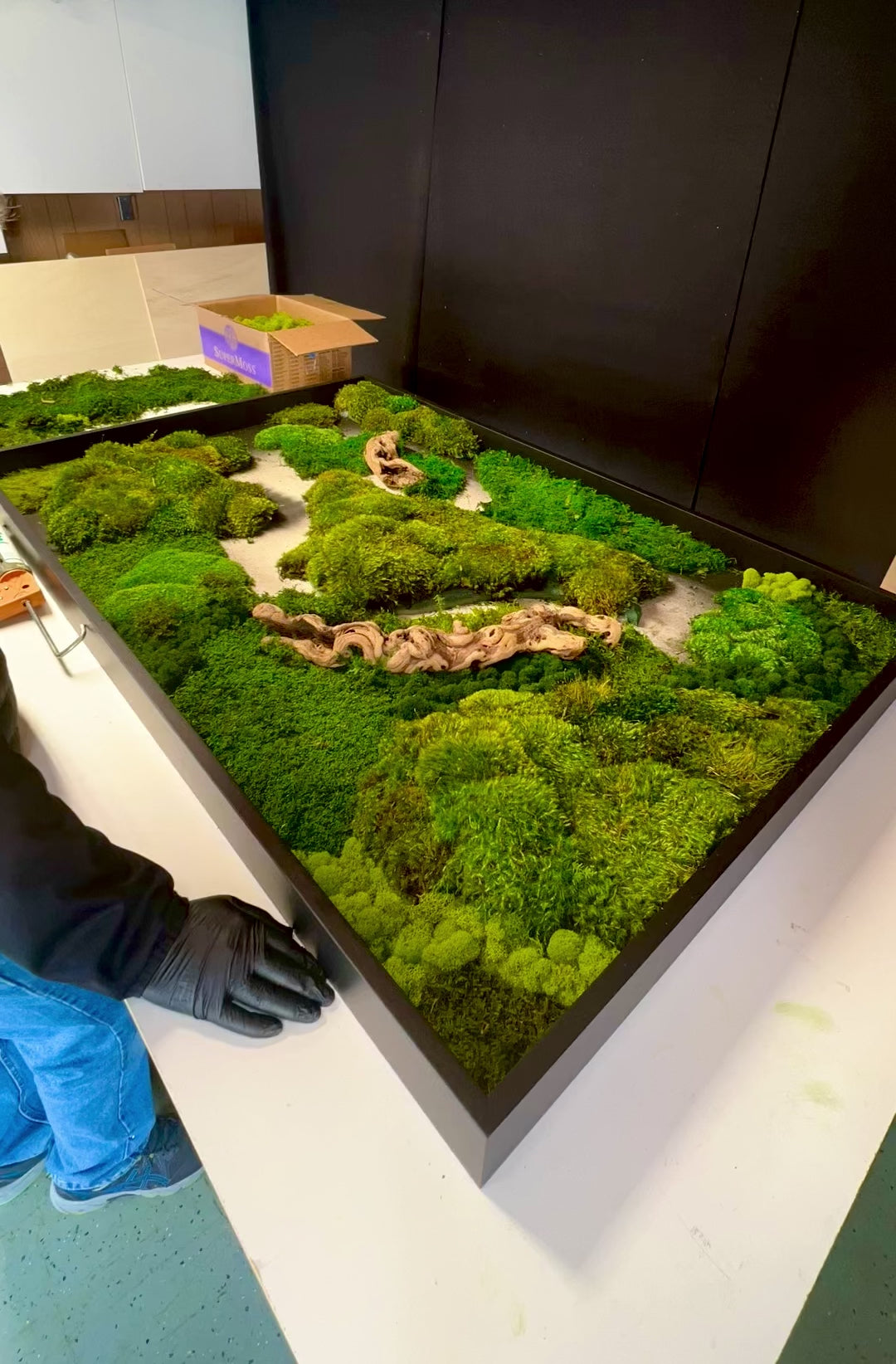The image is a detailed, color photograph capturing a diorama in progress, positioned on a broad, low white table. The diorama itself is a large wooden tray framed in black, giving the impression of a miniature, forested landscape viewed from above. It features meticulously arranged fake plants that resemble little moss piles, with intertwining burl wood branches suggesting driftwood ridges or mountain slopes. 

In the center of the scene, there's a sandy trail flanked by lush greenery, which could either serve as a path or be filled later with fake water to simulate a river meandering through a forest. Around the diorama, various elements are in different stages of assembly: boxes of small, artificial trees lie nearby, along with other vegetation materials and diorama pieces scattered on the table.

A person stands next to the table, partially captured in the left of the frame. They are dressed in blue jeans, flat blue shoes, a long black jacket, and black gloves, seemingly focused on the work. Just visible is the person's gloved hand beside the display, and parts of additional materials are spread out in front of them. Behind the diorama, a tall black structure extends upward, possibly the hinged lid of the diorama case designed to protect and transport the miniature scene. 

The floor of the room displays a gray hue with blue flecks, adding a subtle texture to the setting. Overall, the image depicts a detailed and intricate process of constructing a miniature model, rich in plant life and rock formations, possibly intended to become an elaborate model train landscape or a Japanese garden scene.